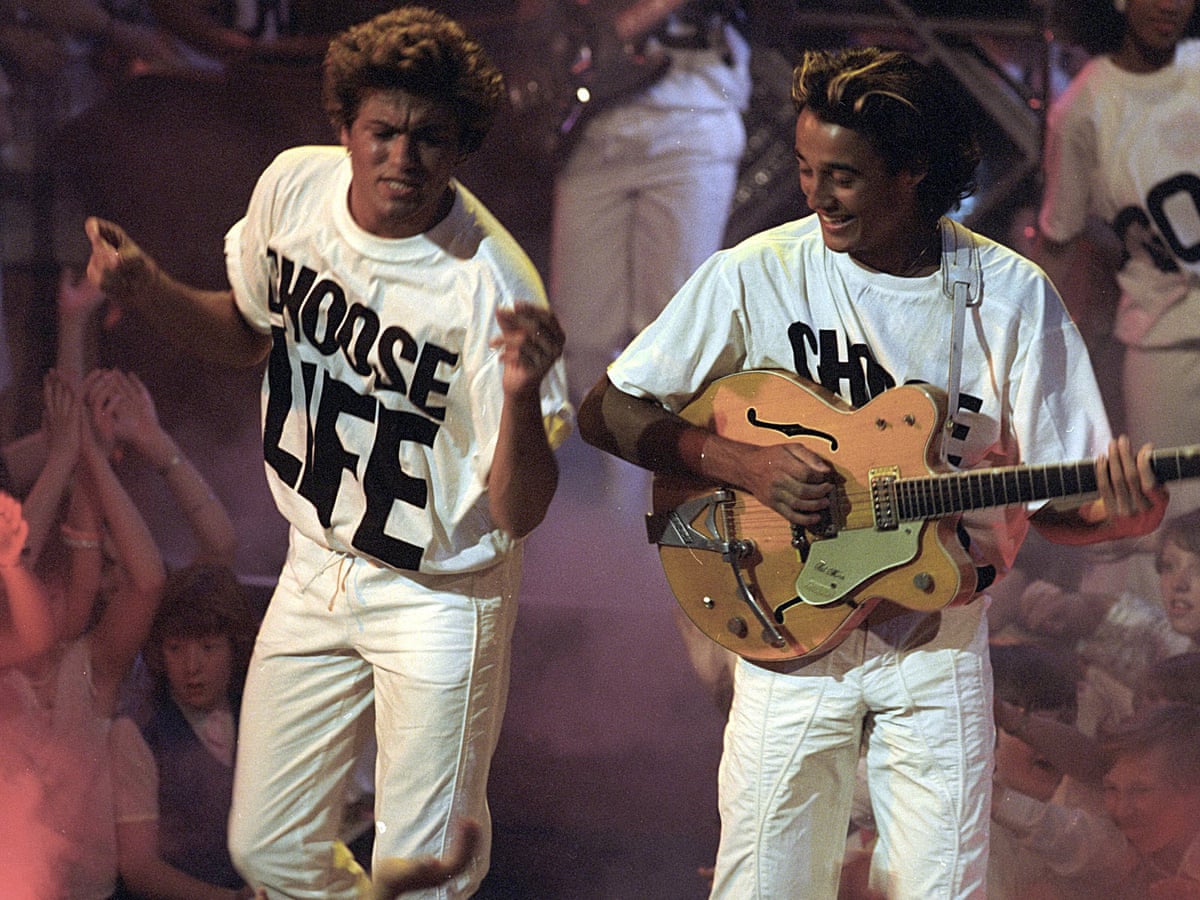This photograph captures the iconic 1980s band Wham during a dynamic live performance. Front and center, we see the band's two male members, George Michael on the left and his bandmate on the right, both dressed in baggy white T-shirts emblazoned with the bold slogan "Choose Life" in black letters, paired with matching white drawstring pants. George Michael, with his curly brown hair, snaps his fingers mid-song while looking into the distance. His bandmate, smiling and engaged, plays a Les Paul Gibson guitar with a wooden body, his wavy dark brown hair highlighted with blonde streaks catching the light. 

In the background, other members of the band, similarly dressed in white attire, provide instrumental support, while the stage itself is cloaked in concert mist. The stage is designed to extend into the audience, creating an immersive experience for the concertgoers flanking the musicians on either side. The enthusiastic crowd, sitting and cheering, adds to the lively atmosphere of the performance. This image encapsulates a vibrant moment from Wham's energetic live concerts, highlighting their charismatic stage presence and connection with the audience.